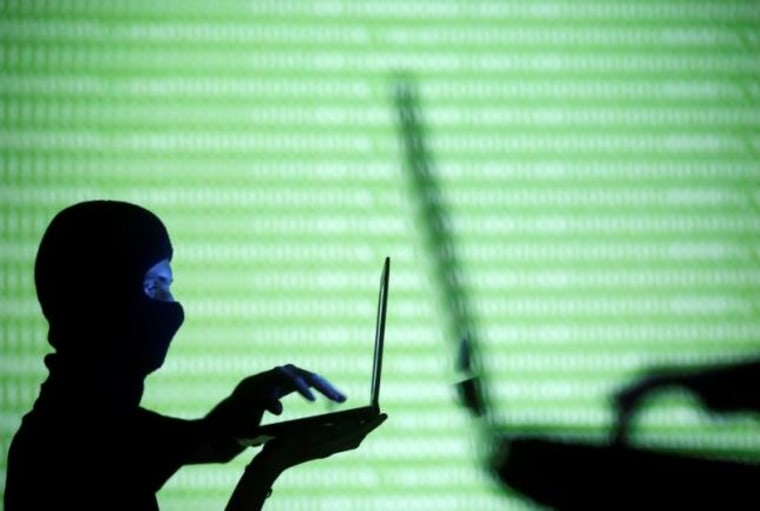This image features a man positioned in the bottom left corner, dressed in all black, including a ski mask that reveals only his eyes and the area just above his eyebrows. The ski mask covers his entire head, emphasizing a sense of anonymity. The man holds a laptop in his right hand while his left hand hovers over the keyboard, poised as if typing. He is dressed in a black long-sleeve shirt, enhancing the ominous, clandestine appearance. The background is a stark, bright lime green interspersed with blurry binary code (zeros and ones), adding a technical, cybernetic atmosphere to the scene. To the right, there is a mysterious shadow of the man and his laptop, flipped in the opposite direction, suggesting a duality or reflection—potentially symbolizing the hidden nature of cyber activities. Overall, the scene evokes themes of hacking and information security.